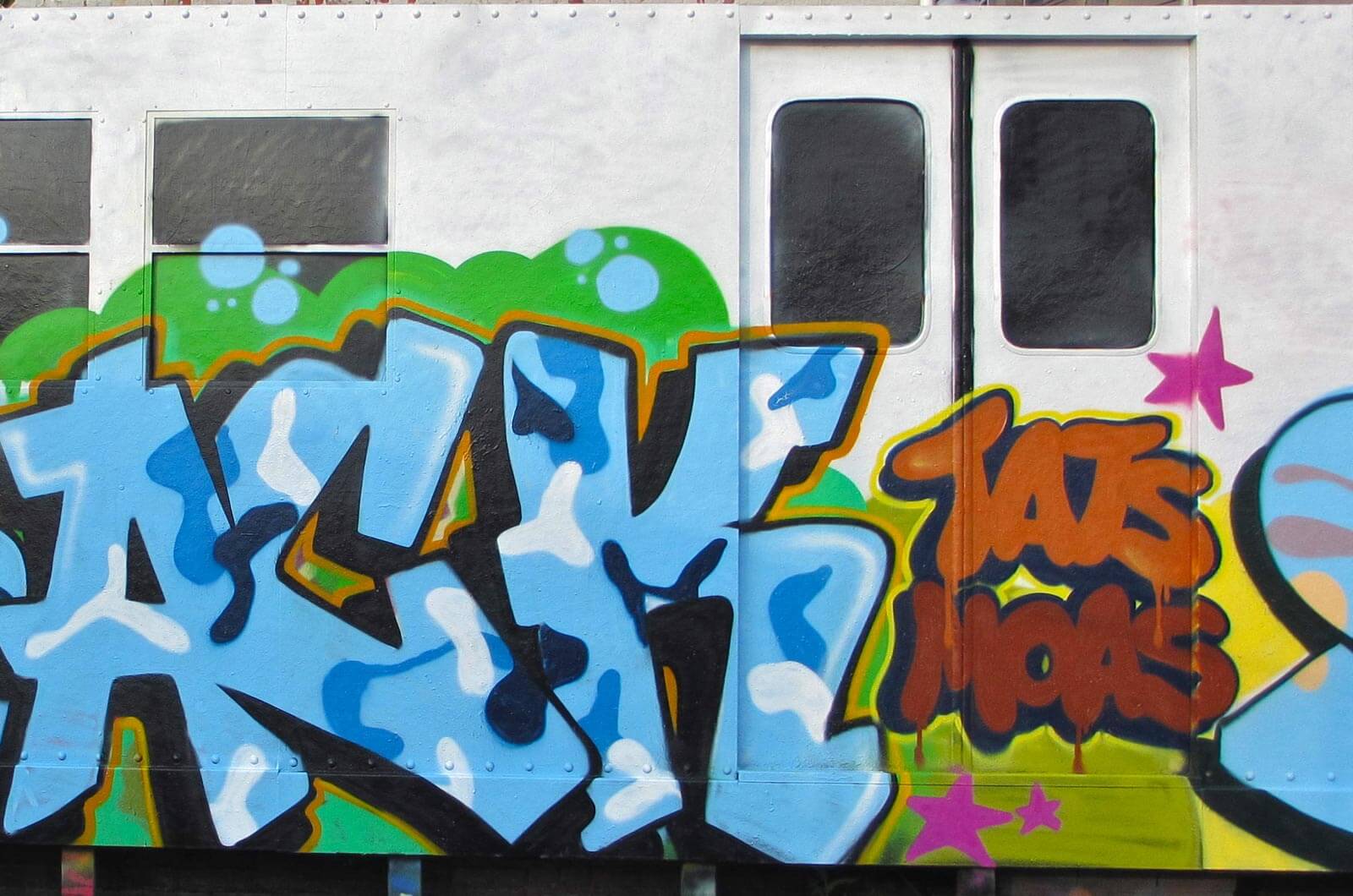This image showcases the side of a light gray subway car adorned with vibrant graffiti. The subway car features a closed set of doors with tinted windows in the upper third, and a couple of additional dark-tinted windows along the side. The car's surface includes evenly spaced steel rivets along the top edge. Dominating the scene, the graffiti is rendered in various vivid hues. The prominent text in graffiti style reads "ACK" in bubble letters, filled with a gradient of white, light blue, deeper blue, and navy blue, all outlined in dark navy blue with an orange border. Behind this main text, a green background color enhances the visual impact. On the right side, the words "TATS" and "MOAS" appear in smaller letters, with "TATS" in orange and "MOAS" in maroon. The artwork is further embellished with pink stars, creating a dynamic and colorful display. The paint spans across the windows and doors, integrating the entire composition into a cohesive piece of urban art.